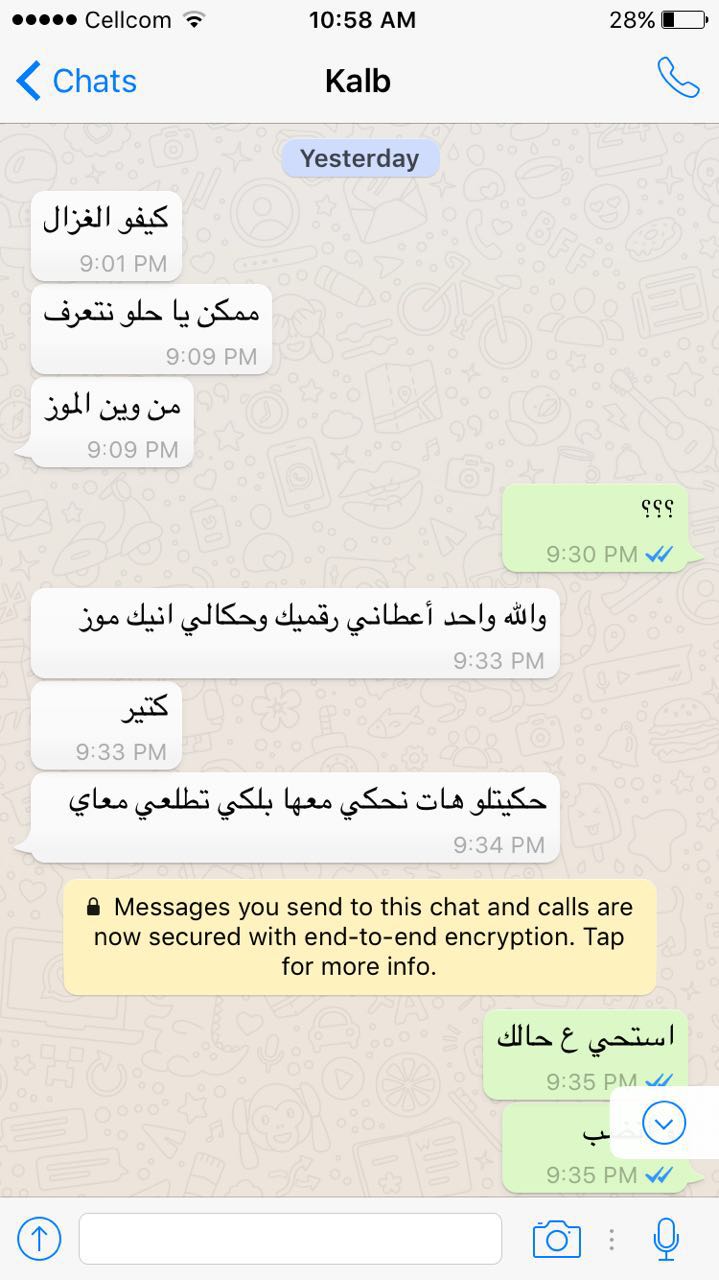This image is a detailed screenshot of a chat conversation on a cell phone with a light blue background. At the very top, a white banner displays the time, battery charge, and the name "CALB" in black, with "CHATS" in blue on the left and a phone symbol on the right. Immediately below, a small blue banner with grey text reads "Yesterday." 

The conversation consists of multiple text exchanges, predominantly in Arabic. On the left side, the timestamps for each message are in a white area—starting with one at 9:01 PM, followed by two more at 9:09 PM. On the right side, green chat bubbles appear with Arabic text time-stamped at 9:30 PM, followed by another message which also includes the text "check check" in blue. 

Further down, the left side continues with white chat bubbles containing Arabic text sent at 9:33 PM and another at 9:34 PM. A notable notification in a pink box with black writing reads, "Messages you send to this chat and calls are now secure with end-to-end encryption. Tap for more info." 

Below this, another blue chat bubble with Arabic text is time-stamped at 9:35 PM, and there is an icon resembling a clock also at 9:35 PM. Navigation buttons are visibly placed at the bottom of the phone screen.